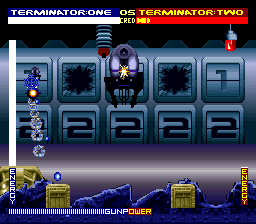The image is a detailed screenshot of a video game, seemingly featuring a scene from "Terminator." At the top of the screen, the left side displays "Terminator 1" in white text against a blue background, while the right side shows "Terminator 2" in yellow text on a red background. Each opponent has a corresponding energy meter below their name: a white bar full for Terminator 1 and a full red bar for Terminator 2. The gameplay involves a gridded area with five rows of squares, where the top row contains various symbols, including a chain-like icon, an obscure hole, a spider, another hole, and a number '1'. The bottom row, on the other hand, contains squares all marked with the number '2'. The layout also hints at a mountainous and watery structure, possibly indicating the in-game environment. The overall theme suggests a metallic blue and purplish color scheme, with a notable feature in the center that appears to be a gun barrel pointing towards the viewer, emphasizing the game's action-oriented focus. Additionally, text at the bottom reads "Gun Peak Power and Energy," which might relate to the game's mechanics or current status.